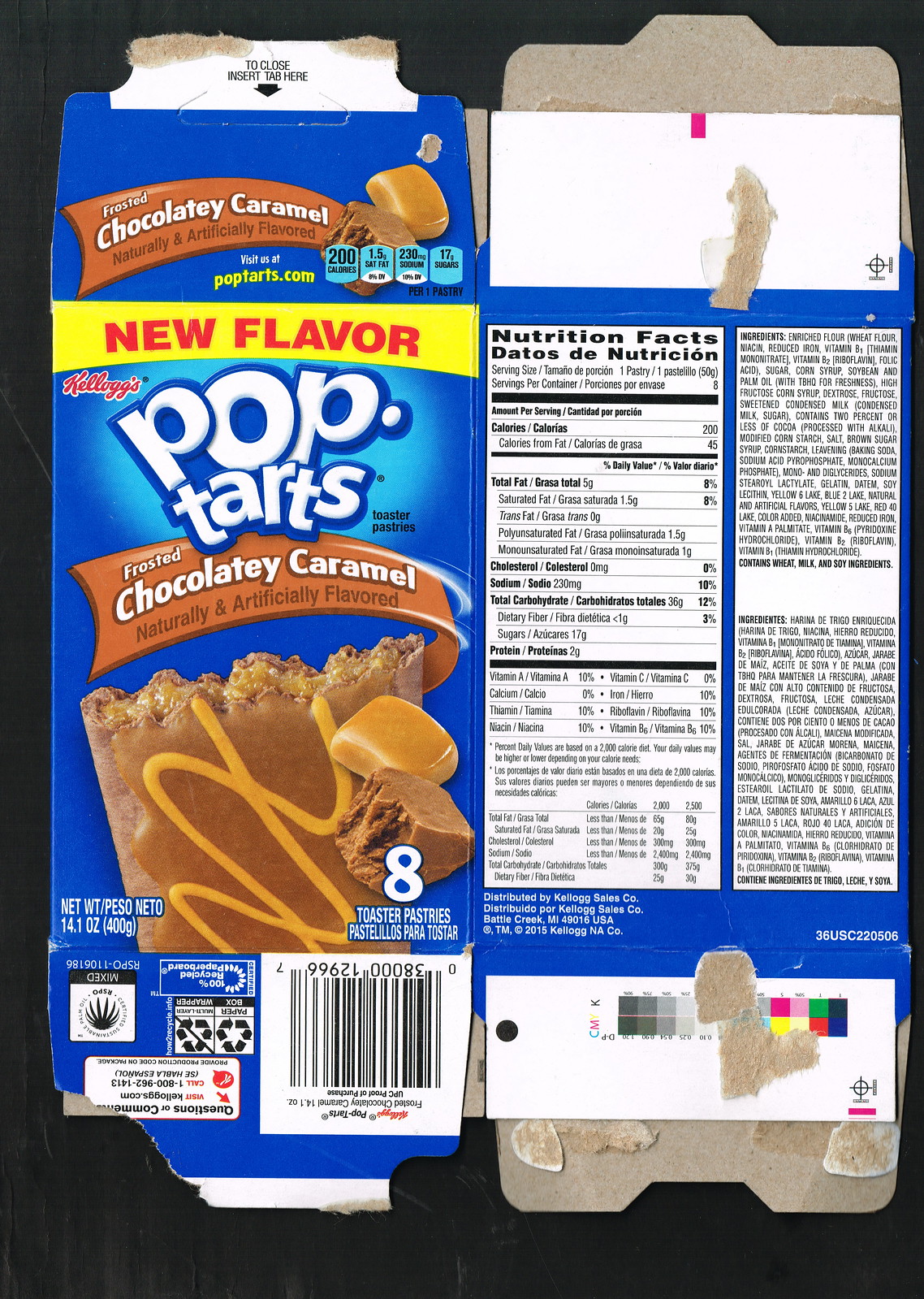This photograph showcases a flattened Pop-Tarts box positioned on a black surface. The box, crafted from thin, blue-colored cardboard, highlights the product's flavor in a prominent brown banner that reads "Frosted Chocolatey Caramel, Naturally and Artificially Flavored." A close-up image of the actual Pop-Tart is also prominently displayed beneath the flavor description. On the rear side of the box, a white panel details the nutrition facts and another white section lists the ingredients. The bottom flap of the box features a white bar containing a black UPC code, recycling information, and a section for customer inquiries directed to the company.